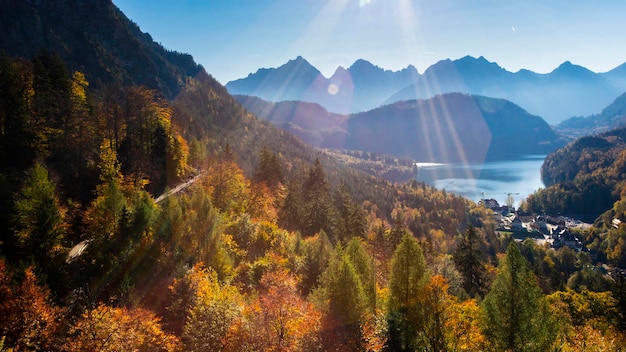This image captures a picturesque mountainside during the fall season, with a vibrant mix of orange, gold, and green foliage, predominantly from evergreen trees. The mountains dominate the left side of the image, while a smaller section appears on the right. In the background, a serene blue body of water stretches out, separating the foreground from a series of more distant mountain peaks that transition from smooth to jagged. The sky above is light blue with rays of sunlight streaming down, suggesting it is a sunny day, possibly taken through a window as there is a faint reflection of the photographer. In the bottom right of the image, a small town or village nestles in a clearing along the edge of a river cove. The landscape features a road running along the mountain's side, emphasizing the elevation from which the photo was taken. This bright and sunny scene encapsulates the tranquil beauty of autumn in a mountainous region.